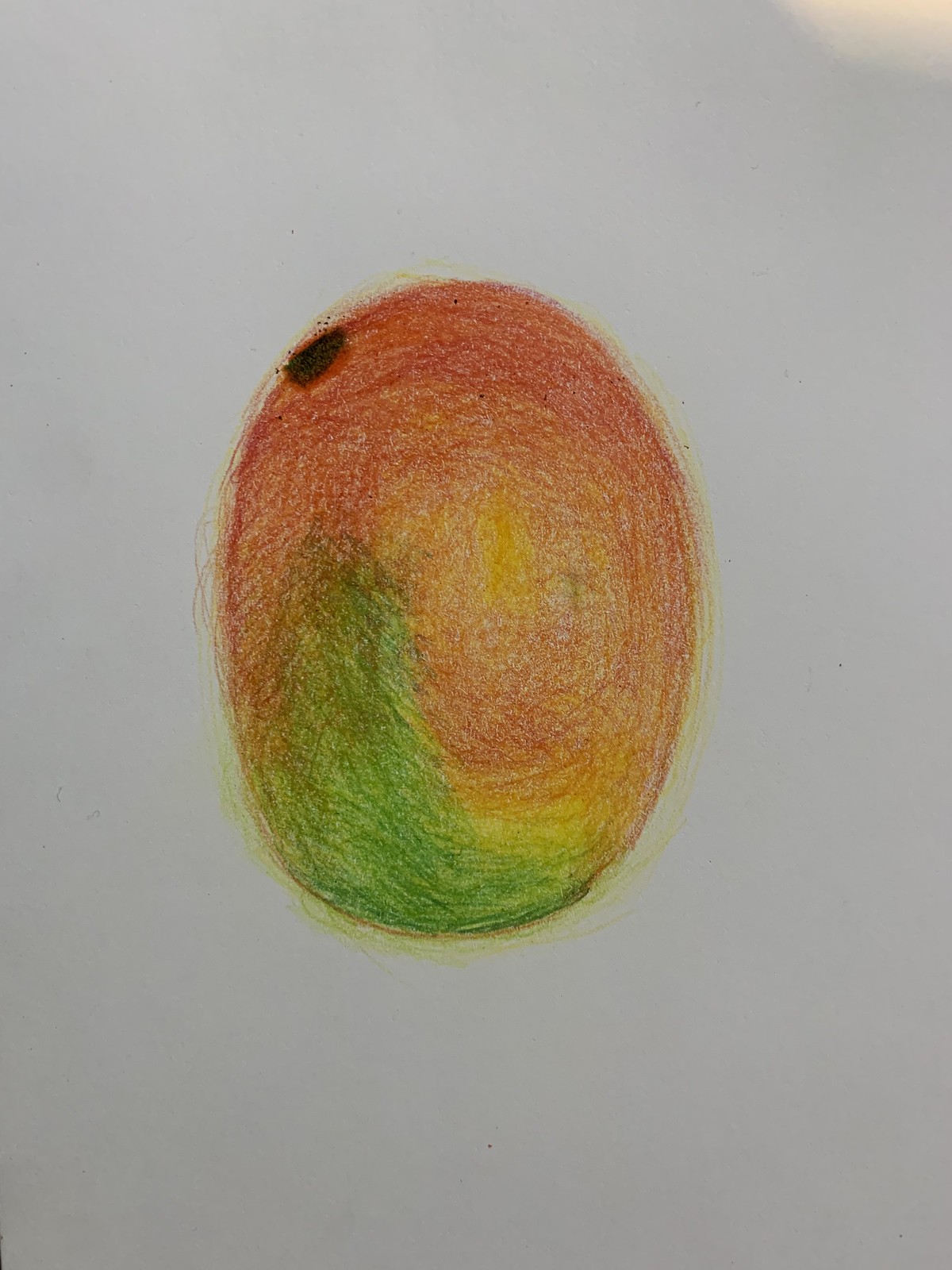The drawing depicts a predominantly orange mango, positioned vertically on a sheet of white paper. The mango is illustrated with a rich array of hues, transitioning smoothly between shades of red, yellow, and orange to capture the fruit's natural gradients. A notable dark red, almost black, spot is present near the top left, possibly representing a bruise. Towards the bottom left, a green swoop suggests the mango is not fully ripe, a common characteristic in both partially ripe and some mature mangoes. Overall, the drawing is simple yet effectively conveys the distinct features of the fruit.